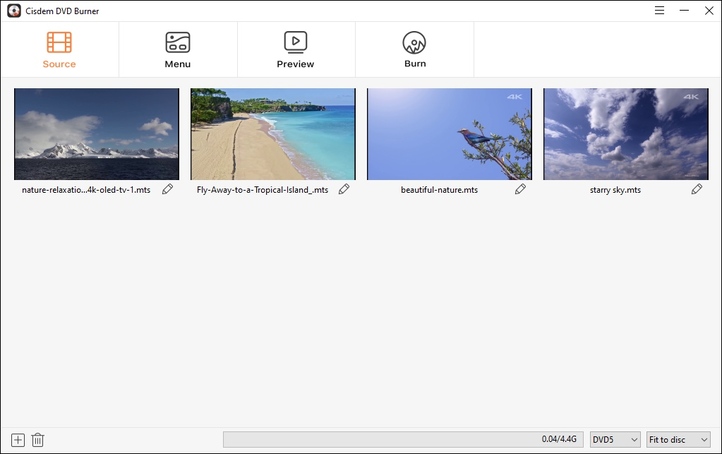This image captures a screenshot from a DVD burning software interface named "System DVD Burner". At the top of the interface, there is a small disc icon with the label "System DVD Burner". The interface features various functional icons, including "Source", "Menu", "Preview", and "Burn" scattered across the screen, which likely correspond to different steps or features within the program.

In the upper right corner are three horizontal lines representing a menu, along with minimize and close buttons. The main section of the interface showcases four distinct images ready for burning: a snowy mountain adjacent to an ocean, a tropical beach, a tree with a bird perched on it, and a sky filled with clouds. 

At the bottom of the interface, additional controls include a trash can icon for deleting items and a plus icon for adding new items. There is also a progress bar indicating space usage, showing "0.04 out of 4.4 GB". Adjacent to this, there are options labeled "DVD 5" and "Fit to Disc", likely representing different output formats or compression options for the burning process.